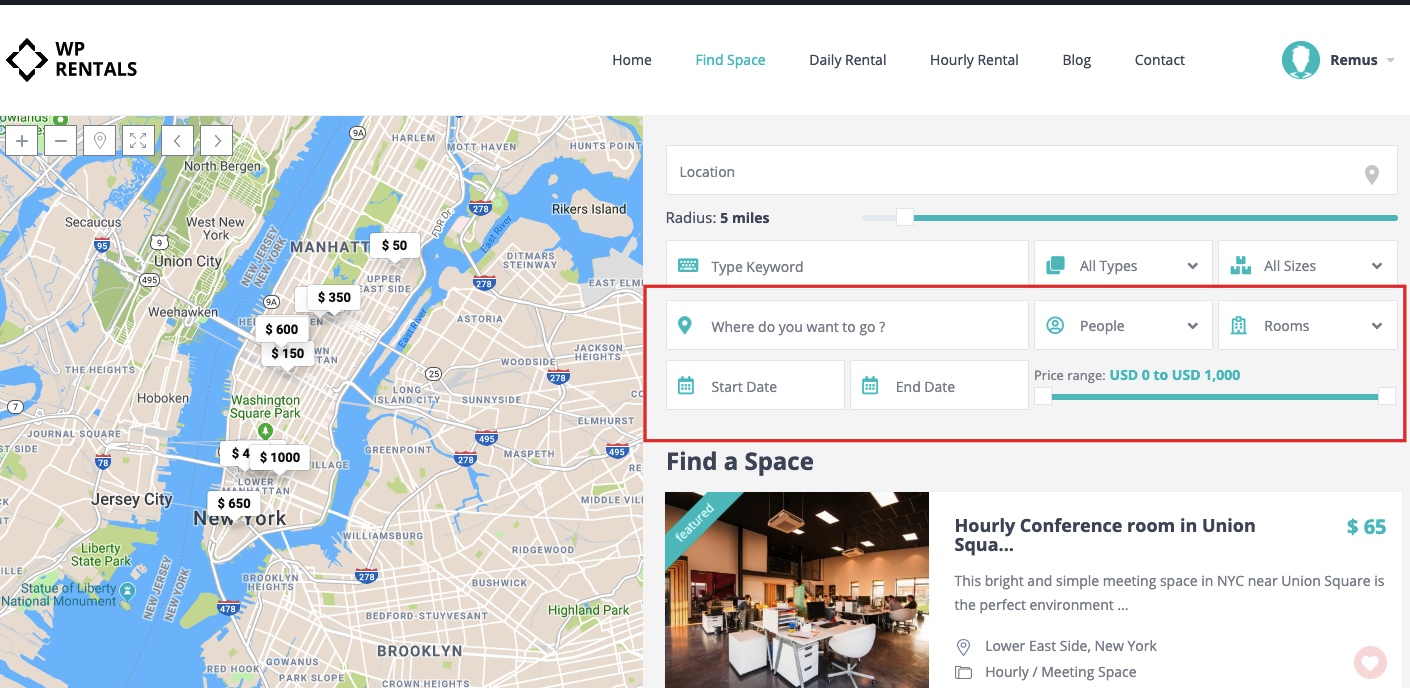The image is a screenshot from the WP Rentals website, displaying a detailed map of New York City, including Manhattan, Brooklyn, Jersey City, Rikers Island, and the Hudson River. The map features interactive zoom buttons marked with plus and minus signs, allowing users to zoom in and out. Overlaying the map are white speech bubble-shaped icons indicating rental prices such as $50, $150, $350, $600, and $1,000. 

At the top of the page, a navigation bar features options like Home, Find Space, Daily Rental, Hourly Rental, Blog, and Contact. On the right side, there is a user profile section labeled “Remus” with a cartoonish profile picture. 

The page highlights the "Find Space" feature, showing search criteria including a 5-mile radius, destination options, number of people, types and sizes of rooms, and keyword search. The date selection includes a start and end date for the rental period. Notably, there is an hourly conference room available in Union Square for $65.